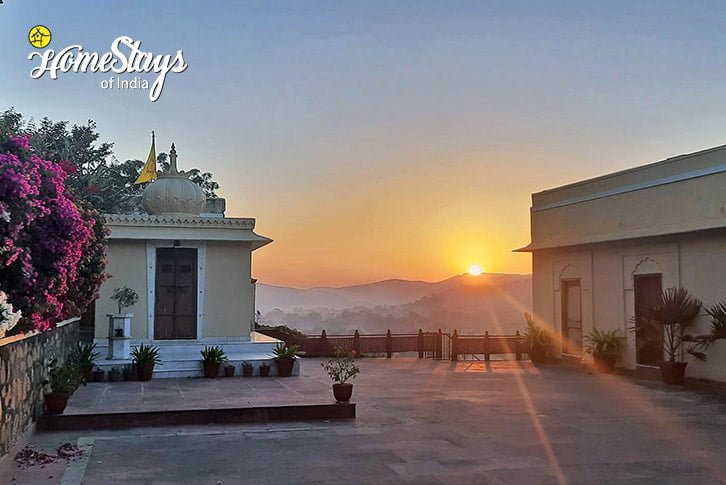This image captures a stunning sunset over a distant mountain range, with the Sun about to dip below the jagged peaks. Rays of sunlight pierce through the sky, casting a golden hue over the scenery. In the foreground, there are two distinct buildings surrounded by lush vegetation and a brown patio fence. On the left, a small tan-colored building displays ornate, Indian-style architectural details and has a brown door. Above it, text reads "Homestays of India," accompanied by a yellow circle outlined in black, featuring a small black house. To the right, part of a longer building is visible, also with a brown door and encircled by numerous plants. A stone wall adorned with bushes, including one with vibrant pink flowers, adds to the picturesque setting. Adjacent to the buildings, greenery flourishes, enhancing the serene, palatial ambiance of this outdoor space.